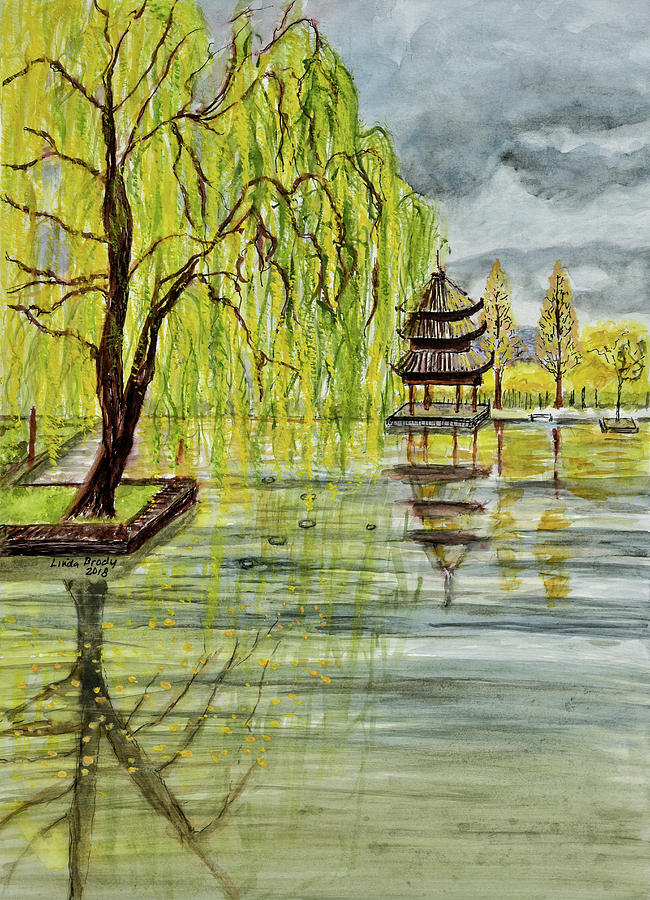This rectangular watercolor painting, measuring approximately six inches high by three inches wide, depicts an exquisitely tranquil and peaceful scene created by Linda Brady in 2018, as indicated by her small signature in black text. Dominated by blue, green, and yellow hues, the artwork features a calm, reflective body of water, likely a lake or large pond, devoid of waves and crystal clear. On the left side, a large, dark brown willow tree with long hanging vines of golden yellow and green leaves leans over the water, its reflection mirrored on the lake's serene surface. Midway through the painting, in the background, there's an oriental-style building with three distinctive roofs, raised on stilts, evoking an Asian-inspired architectural aesthetic. Adjacent to this structure, more trees covered in yellow autumnal leaves add to the scene's natural charm. The sky is depicted in varying shades of gray, suggesting a dark and gloomy atmosphere, yet the overall composition of the painting remains beautiful and meditative.